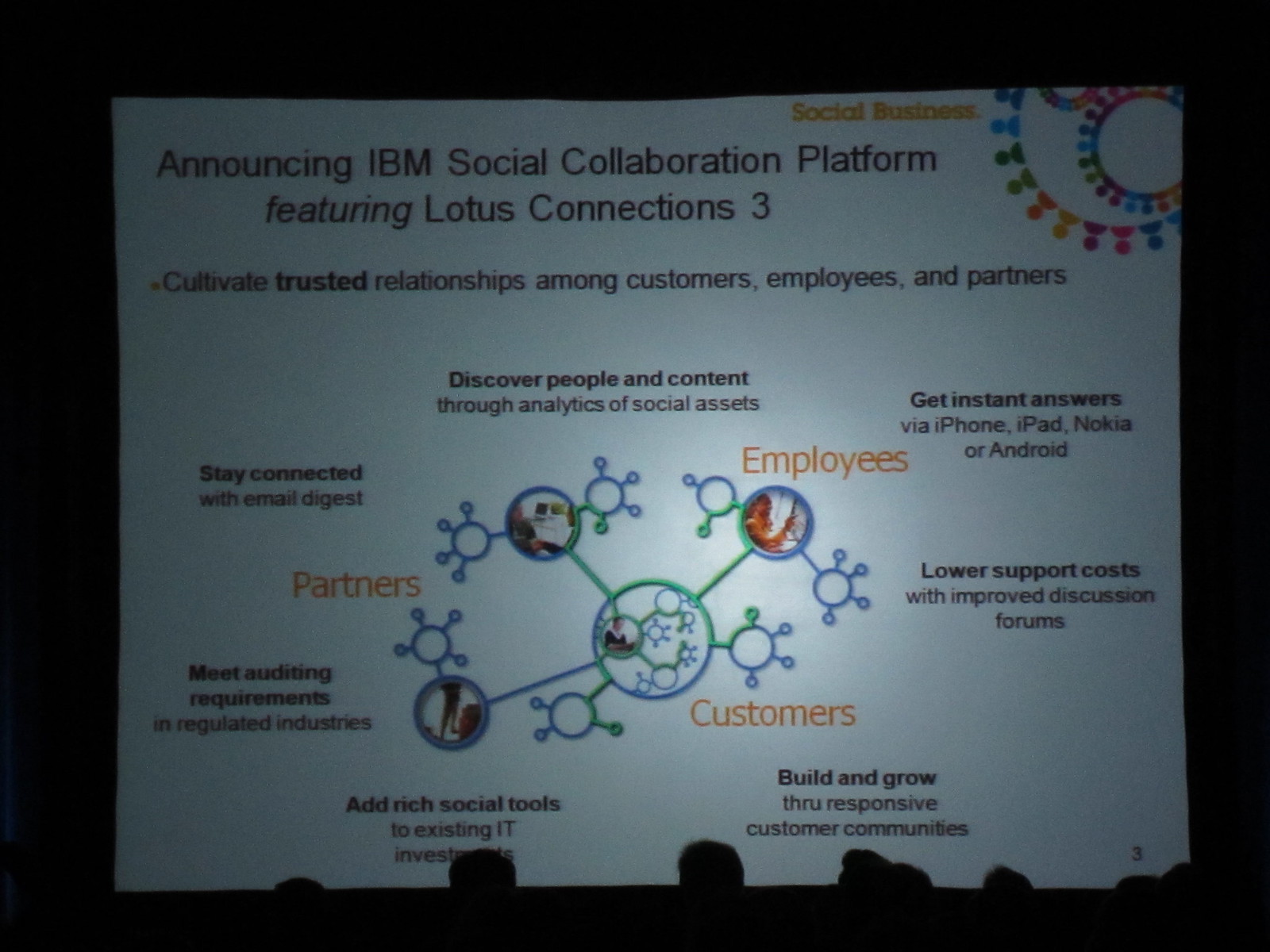This detailed and descriptive caption captures the essence of the shared elements with emphasis on what's repeated across the different descriptions:

---

Taken from the perspective of an audience in a darkened room, this photograph shows the silhouettes of several people against a large, illuminated slide. The white slide features black text under the headline, "Announcing IBM Social Collaboration Platform Featuring Lotus Connections 3," with "Social Business" emblazoned in orange text at the top right. The presentation outlines the platform’s core goal: "Cultivate Trusted Relationships Among Customers, Employees, and Partners." Surrounding a central diagram of interconnected circles – with blue and green lines linking blue dots of varying sizes – are details on the platform's capabilities. Key features include discovering people and content through social analytics, getting instant answers on various devices (iPhone, iPad, Nokia, Android), lowering support costs with improved discussion forums, building and growing customer communities, adding rich social tools to existing IT investments, meeting auditing requirements, and staying connected with email digests. The network diagram emphasizes three primary nodes: Partners, Customers, and Employees. Outlined human heads are visible along the bottom of the image, further highlighting the collaborative focus of the platform.